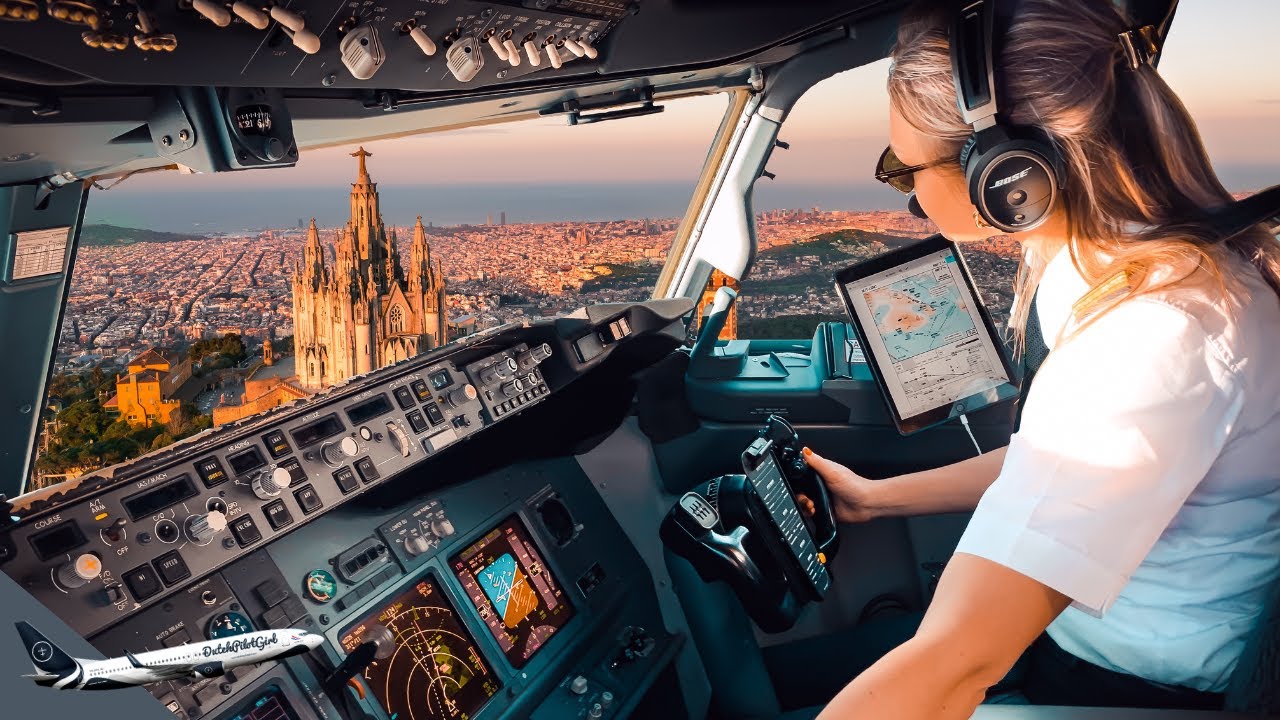This detailed image, presumably AI-generated or photoshopped, captures the interior of an airplane cockpit piloted by a young woman. She is wearing Bose headphones and a white top with a blue gradient that extends downwards, paired with black pants. A microphone is positioned next to her face. The pilot has her right hand on the yoke-style steering wheel or stick, possibly aiding in controlling the plane.

In front of her lies a complex instrument cluster with numerous switches, lights, knobs, and dials, along with an iPad plugged in and mounted to the right of the cockpit. Above the instrument cluster is a compass, central to her view. Numerous switches are also visible above her.

Through the cockpit window, the scenic view of Barcelona is juxtaposed with the landscape of France, especially highlighting the Notre Dame cathedral. Additionally, clusters of housing and greenery complete the picturesque aerial scene. Illuminating the branding "Dutch Pilot Girl," this image suggests a promotional or entertainment material, framing a serene yet detailed moment of piloting amidst a significant urban and natural panorama below.